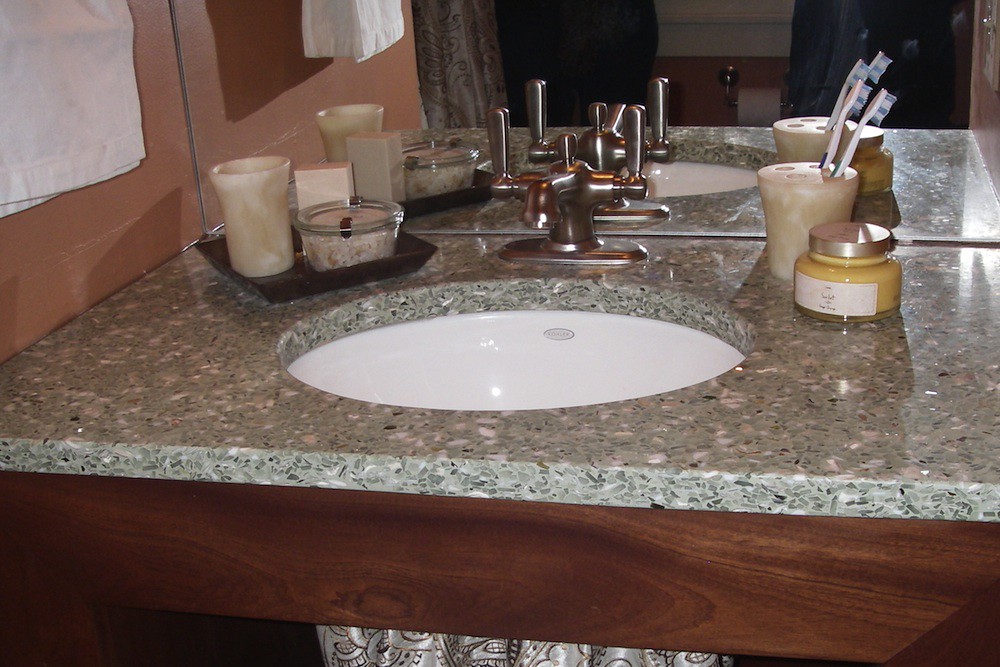This photograph showcases a modern bathroom sink with intricate details. The sink itself features a striking marble texture in shades of gray, green, and white, set atop a sturdy wooden frame. The basin of the sink is a clean, crisp white, creating a pleasing contrast with the marble surface. A metallic faucet with sleek, upward-facing handles for hot and cold water sits on top of the sink, adding a contemporary touch.

On the right side of the image, there is a yellowish-white toothbrush holder with four holes, housing two white toothbrushes adorned with blue bristles. In front of the holder, closer to the viewer, stands a glass container filled with a yellow substance, sealed with a metallic lid and labeled with a small white rectangular sticker, though the text remains indistinguishable.

To the left of the sink, a black tray displays three distinctively shaped candles: a short circular candle, a tall cylindrical one, and a medium-height cube candle. The tallest candle boasts a yellowish hue, while the other two express more subtle, faded pink tones. 

At the far end of the sink, a mirror reflects the scene, set against a salmon-colored wall. A white towel hangs from the left side, aligning with the wall and completing the composition. This detailed arrangement offers a harmonious blend of colors and textures, accentuating the modern aesthetics of the bathroom.